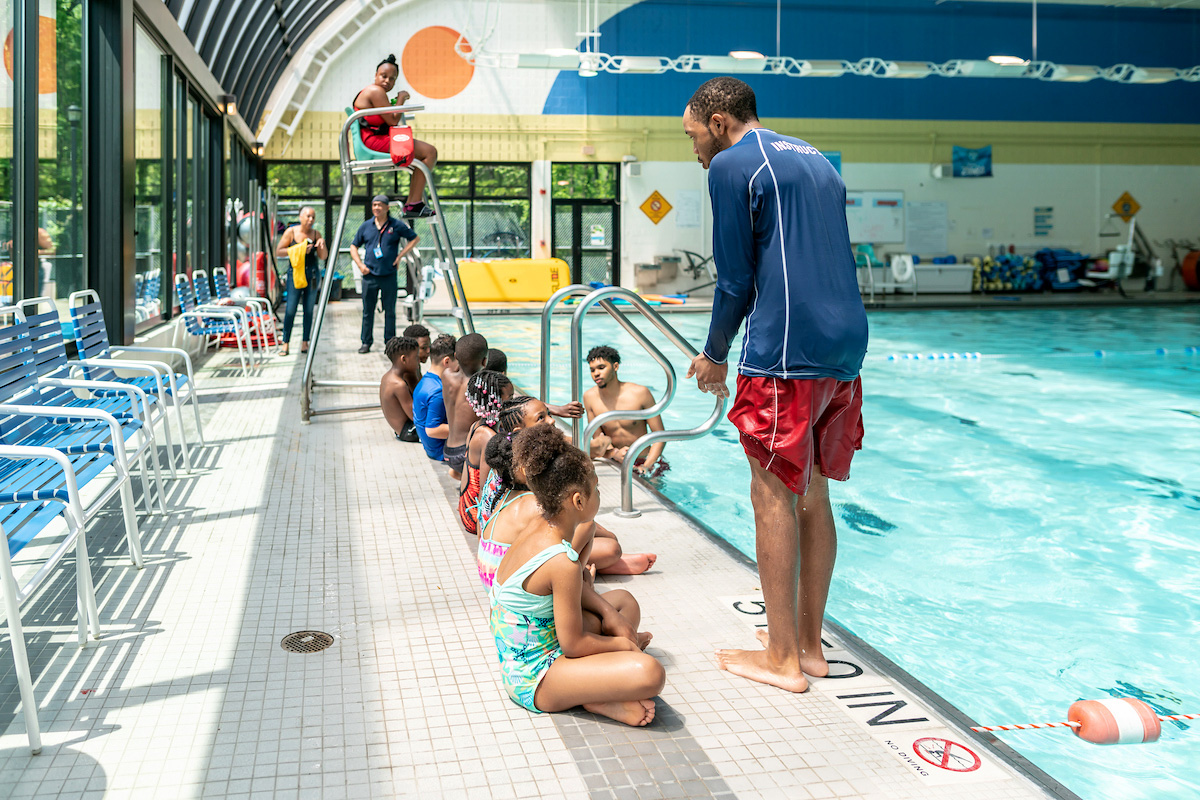This vibrant image captures the dynamic environment of an indoor community pool bathed in bright sunlight streaming through floor-to-ceiling windows, framed with black bars at regular intervals. The pool area is bustling with activity as a group of approximately a dozen young African American children, seated in a neat row on the white and gray tiled floor beside the pool, attentively follow instructions from a swim coach. The coach, a young African American male dressed in a long-sleeved dark blue rash shirt and red swim trunks, stands at the edge of the crystal-clear light blue water, prepared to guide the children through their swimming lesson. In the mid-ground, a female lifeguard in red attire sits vigilant atop a high lifeguard chair, observing the scene carefully. Flanking her, two other figures stand behind the chair, adding to the scene's sense of supervision and community. The back wall of the pool area is adorned with a cheerful mural featuring a large orange sun, yellow and blue stripes, enhancing the pool's welcoming atmosphere. Blue and white slatted pool chairs line up in front of the large windows, completing this detailed depiction of a lively and well-organized swimming session.